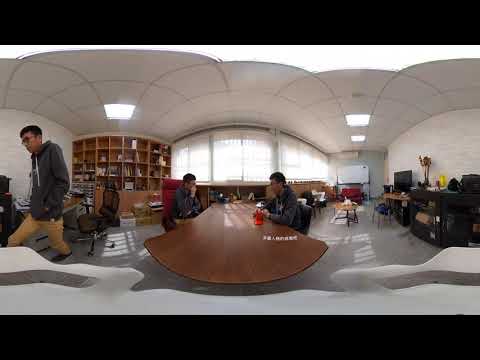In a panoramic 360-degree view of a spacious, indoor room, a long, polished wooden table dominates the center where two Asian men in glasses, both wearing black long-sleeved tops, sit facing each other in serious conversation. Behind them stretches a large window, covered with shades, extending from one side of the room to the other. To the left, a man in a long-sleeved black hoodie and yellow pants walks toward the edge of the frame, where a four-row, multi-column brown bookshelf filled with various items stands in the left corner. On the right side of the image, a black cabinet supports a TV placed on another brown desk, accompanied by several smaller independent desks and an arrangement of chairs scattered throughout the background, reinforcing the academic or corporate atmosphere of this functional workspace.